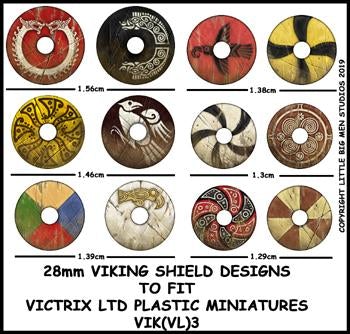The image features a neatly arranged display of 12 miniature Viking shield designs, intended for 28mm Vitrix LTD plastic miniatures. Each shield is circular with a hole in the center, and they vary widely in color and design. The shields are organized into three columns within a square frame. Detailed designs include a red shield adorned with two dragons forming a circular pattern, a black shield with silver engravings covering half, and a yellow shield with intricate black swirls positioned at the noon, six, nine, and three o'clock points. Other shields showcase vibrant combinations of blue, green, red, yellow, and tan. The text at the bottom of the image reads "28mm Viking Shield Designs to fit Vitrix LTD plastic miniatures," highlighting the miniature nature of these decorative pieces.